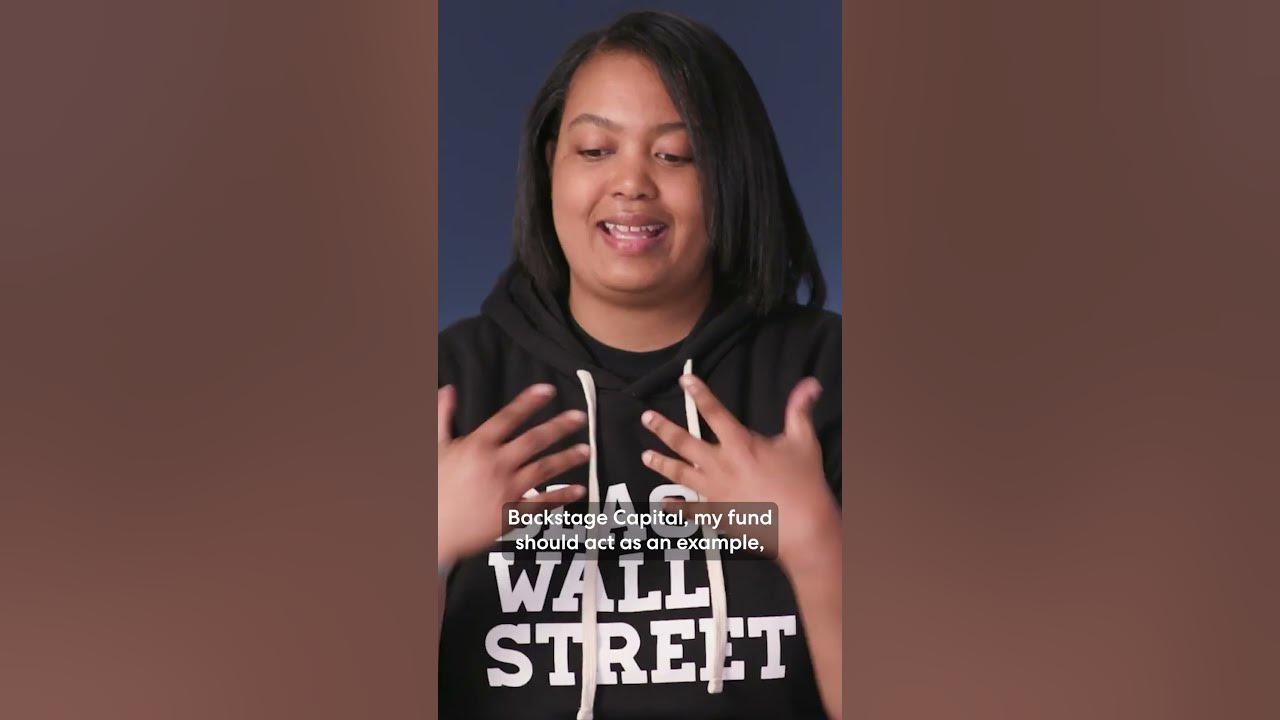The image is a poster likely used for advertisement purposes. The central focus is a woman with long, dark hair against a blue background. She has dark, beautifully brown skin that suggests she might be of African-American or a similar ethnic background. She is wearing a black sweatshirt with white strings, with the visible text "Wall Street" printed on the front—though the first word is obscured by her hands, which are raised and positioned near her chest. She appears to be either in the midst of smiling or talking. The sweatshirt is accompanied by a small, rectangular text box in the middle that reads, "Backstage Capital, my fund should act as an example." The image is framed by two dark brown rectangular areas on the left and right sides, providing a balanced and striking contrast against the bright blue background behind her.